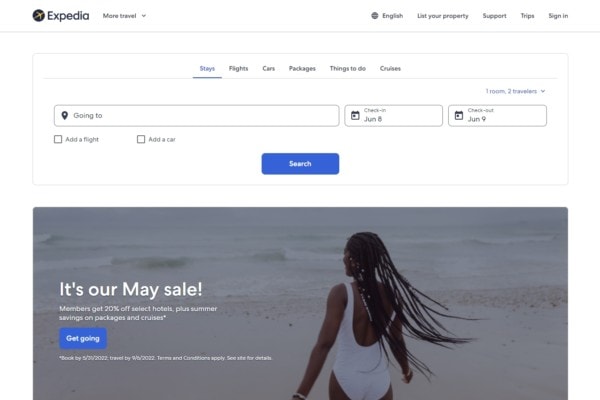The image is a screenshot from the Expedia website. At the top of the page, an airplane icon is visible along with the text "More travel." Adjacent to this, there is a globe icon next to the word "English." The navigation bar includes options such as "List your property," "Support," "Trips," and "Sign in."

Further down the page, a rectangular section presents categories including "Stays," "Flights," "Cars," "Packages," "Things to do," and "Cruises." Below this, there are input fields accompanied by a black map pin icon where users can type in their destination under "Going to." The check-in date is set to June 8th, while the check-out date is June 9th. There are also checkboxes for adding a flight or a car to the booking. Centrally placed on the page, a blue "Search" button invites users to proceed.

At the bottom of the page, there is an image of an African American woman with long braided hair, wearing a white bathing suit and an accessory on her left arm (either a watch or a bracelet). She stands on a beach, approaching the water. The image promotes a sale with the text: "It's our May sale. Members get 20% off select hotels plus summer savings on packages and cruises." Below this text is a clickable blue button labeled "Get going."